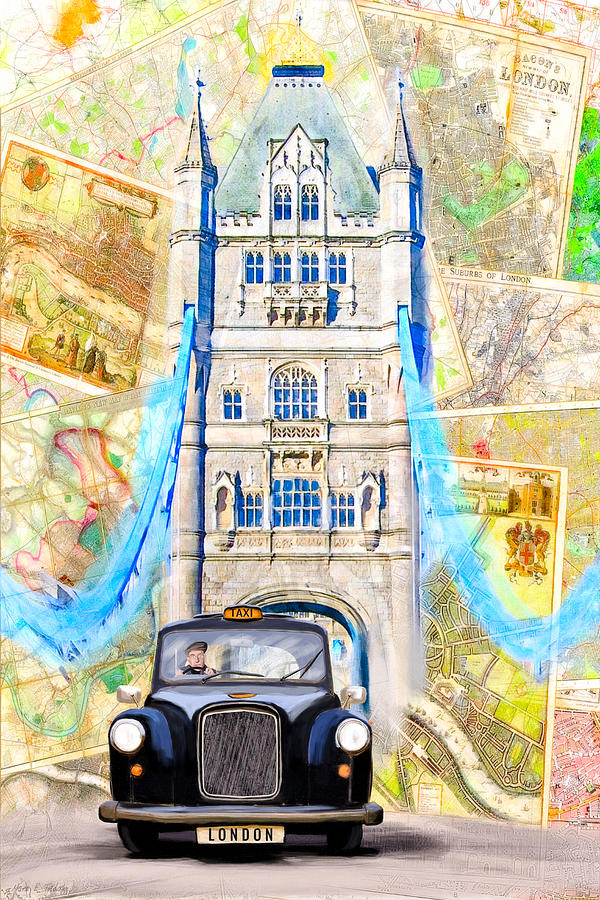This detailed cartoon-style artwork, set outdoors, portrays a vintage English taxi navigating a painted road. The taxi is black with a prominent orange "TAXI" sign above the windshield and a license plate that reads "London." The vehicle features two headlights, a silver metal bumper, and a front grille, with a white man driving from the left-hand side, true to British style.

The backdrop is an intricate collage of brown and orange maps with "Bacon's London" inscribed on one of them. Central to the scene is the Tower of London, a three-story stone building with green gabled roofs and two spires. Blue windows adorn the tower, and vibrant blue ropes appear to bridge the skies behind it. The composition, in portrait mode, creates an elongated effect with these elements weaving together a nostalgic portrayal of London scenery.